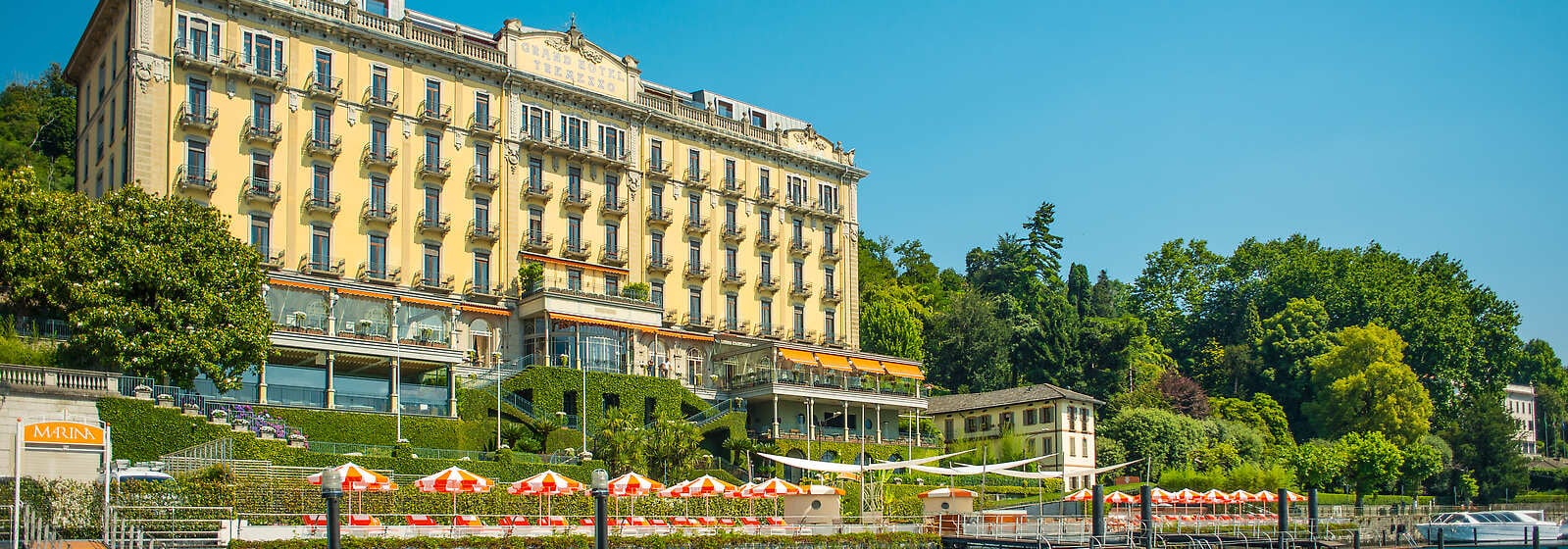The image features a large, grayish-beige rectangular building positioned predominantly on the upper left side. The building appears to have between four to six floors and is partially cut off at the top. A prominent railing traverses the rooftop from left to right, hinting at an accessible rooftop area. In the central facade, an awning juts outward, likely marking the entrance. Below, the setting transitions into a manicured landscape with green hedges and a gentle grassy incline.

In the foreground, a fence runs horizontally from left to right, behind which sits an outdoor seating area filled with red and white umbrellas and matching chairs. This seating area extends across the bottom of the image. The lower left corner reveals a small entryway among the umbrellas and chairs.

On the right side of the image, a copse of various trees dominates the scene, providing a natural contrast to the man-made structure and hinting at a peaceful setting. The sky above these trees is a clear, unbroken blue. Additionally, a glimpse of another building peeks through the trees on the far right bottom edge of the image, suggesting more structures nearby. The overall atmosphere is reminiscent of the front of a grand hotel, with aesthetic similarities to the famous Grand Budapest Hotel from Wes Anderson's film.